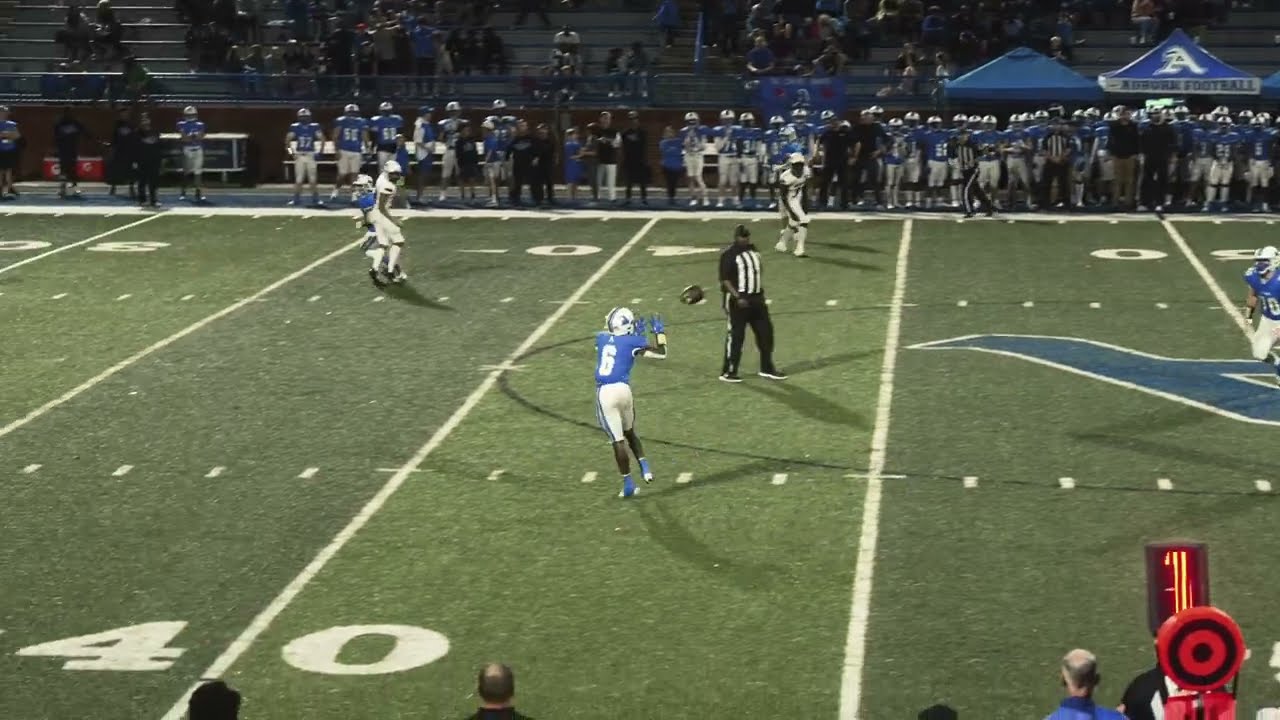This photograph captures an American football game in progress on a green turf field, demarcated by white yard lines. Dominating the midsection of the image, a player in a blue jersey, white pants, and a white helmet is poised to catch a ball suspended in mid-air near the 40-yard line. The scene is supervised by a referee clad in traditional black-and-white stripes, with a black hat and white pants accented by black stripes.

The field is populated by five players and the referee, with additional players and coaching staff standing along the sidelines, observing the action. The players from the opposing team are dressed in all-white uniforms, with some black detailing. An orange down marker and a conspicuous red target, resembling a bullseye, add vibrant touches of color to the field.

Beyond the sidelines, the image extends to the spectator stands, revealing fans seated and watching the game intently. The overall atmosphere suggests a lively high school football match, underscored by the meticulously captured details of uniforms, field markings, and the engaged crowd.